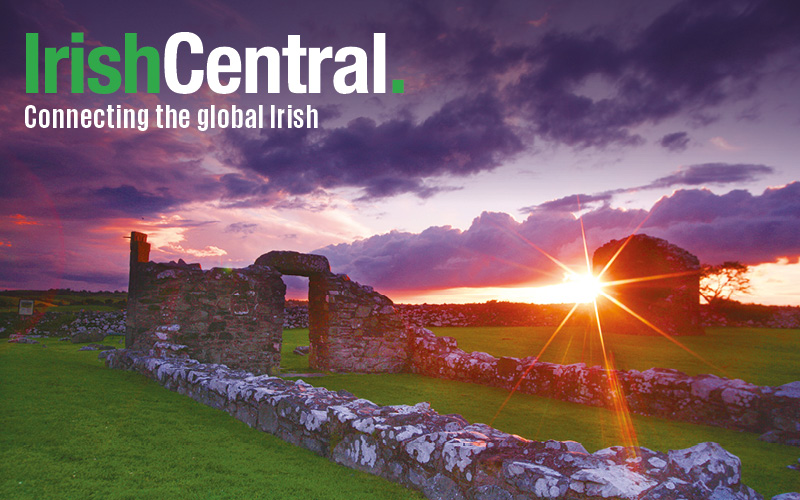A picturesque advertisement set against the backdrop of an ancient stone ruin in a lush, green meadow. The foreground features the remnants of what appears to be the foundation of an old building, constructed from stone and granite, with a distinct archway that suggests a former door. Walls connected by a broken-down row of stones showcase weathered hues of white, earthy red, and brown. In the distance, a horizon of stone fences stretches as far as the eye can see. As the day ends, the setting sun casts a bright orange glare, illuminating the scene with its rays piercing through the horizon. The sky is a dramatic blend of colors—dark purple clouds contrasted by blue sky peeking through, with additional tones of dark pink, orange, and yellow near the horizon. The overall mood is serene, with the silhouettes of trees gently framing the scene. At the top of this advertisement, the company logo "Irish Central" stands out, with "Irish" in green and "Central" in white, followed by a green period and the slogan "Connecting the Global Irish."